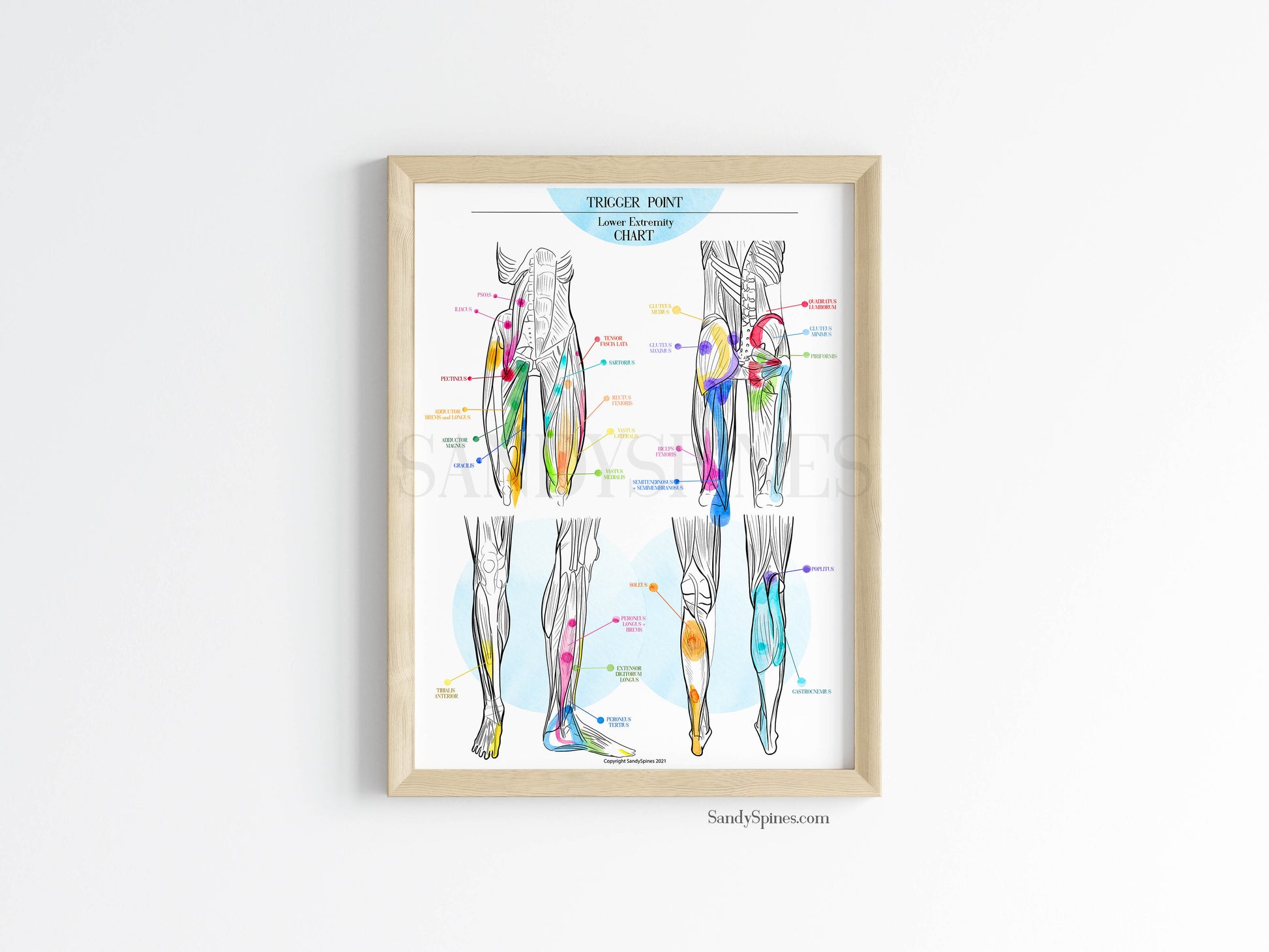This descriptive caption of the image consolidates details from all three voice descriptions, emphasizing shared elements:

The wall-mounted poster, framed in a light tan wood, features a detailed "Trigger Point Lower Extremity Chart." It visually depicts various parts of the lower body, with the primary illustrations showing muscle and bone anatomy from the knees to the ribs. The top of the poster displays the title in black text within a blue semicircle. Each of the four sections highlights specific muscle areas with colored points and corresponding arrows: yellow for the shin, blue for the calf, and other colors like red, green, and orange for additional regions. The images detail both the front and back views of the legs, emphasizing trigger points with labeled bullet points. The bottom of the poster includes the website "SandySpines.com." The entire piece is illuminated from the right, enhancing the visibility of the detailed medical illustrations against the white wall background.